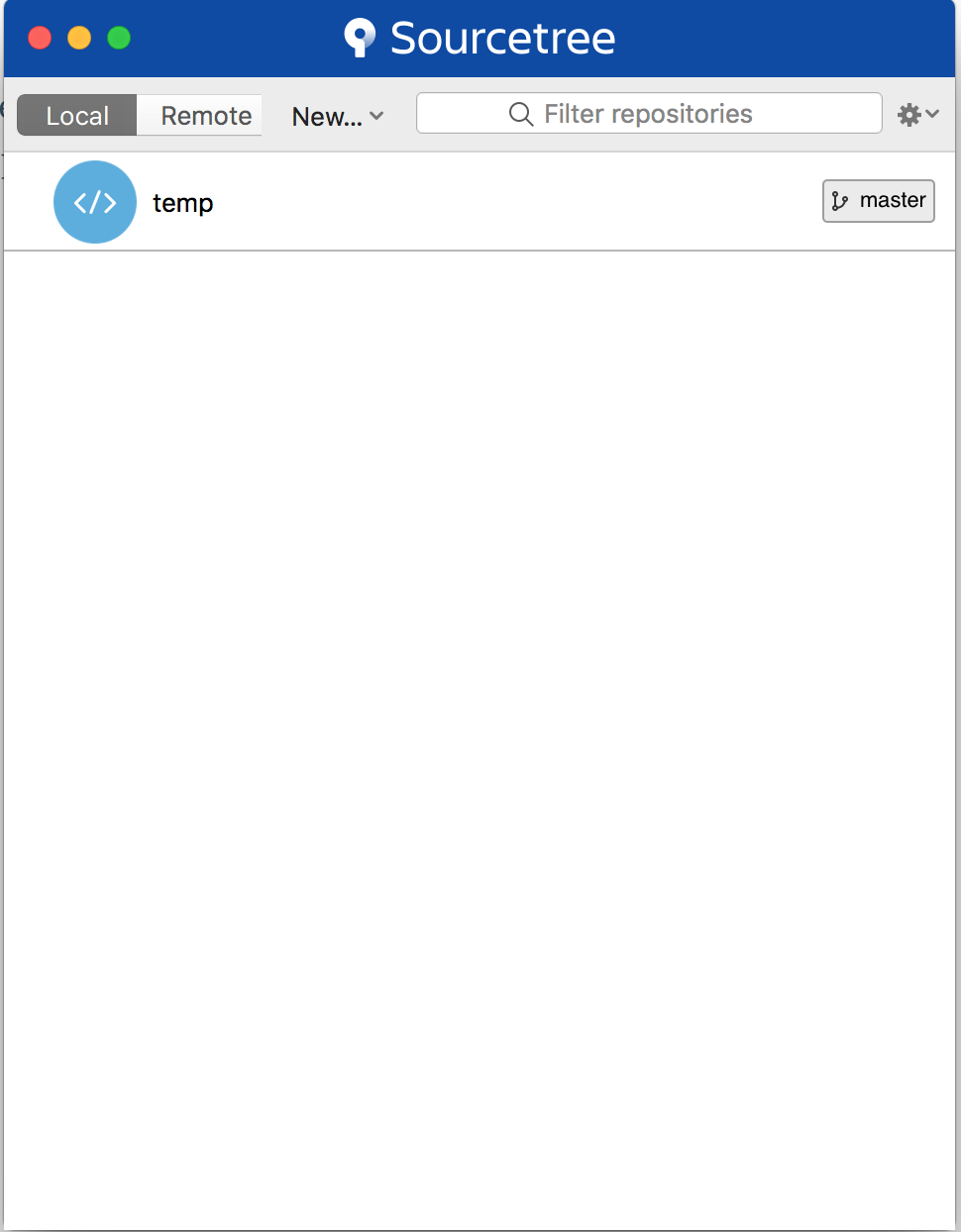The image illustrates a software interface design, prominently featuring a blue rectangle at the top. On the left-hand side of this blue banner, three distinct circles in varying colors—orange, yellow, and green—are displayed, alongside a white symbol. Centralized within this blue section, the text "SOURCETREE" is prominently displayed.

Below the blue section, there is a light gray rectangle followed by a darker gray rectangle with subtly curved corners at the upper and lower left sides. The darker rectangle contains the word "local" in white text. Adjacent to it, another white rectangle reads "remote" and is positioned just below this, featuring a text "new..." along with a downward-pointing arrow.

A white search box outlined in gray, containing a magnifying glass icon, bears the label "filter, repositories." There is also a settings icon with a gear shift symbol and a downward-pointing arrow next to it.

Further down, within a white rectangle outlined in gray, there is a blue circle with an arrow pointing to both the left and right, followed by the text "temp." Close by, a gray rectangle displays three dots connected by lines, labeled "master."

Additionally, another white rectangle outlined in gray remains blank at the bottom right section of the interface.